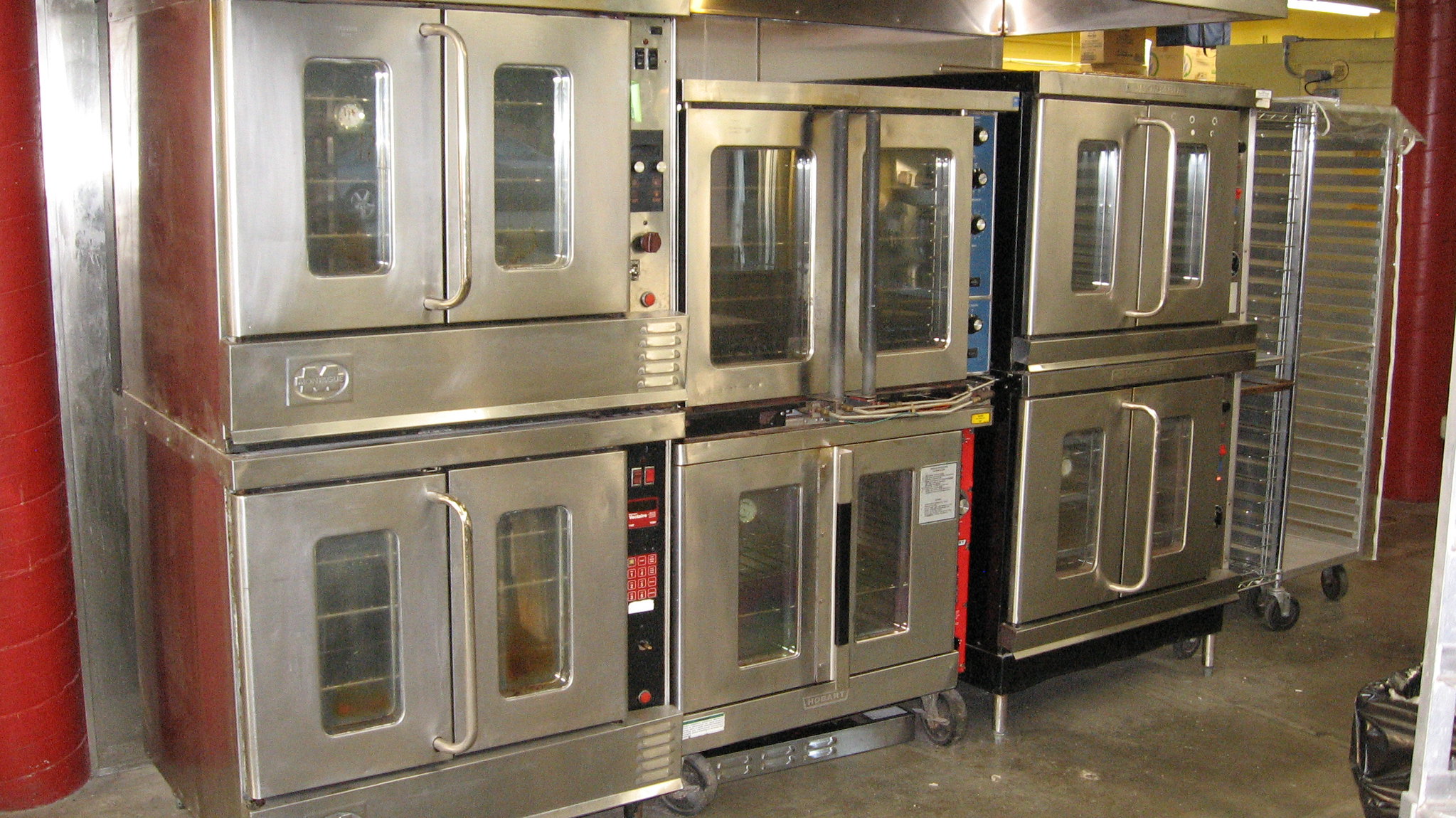The photograph captures a landscape-oriented indoor scene featuring a back wall lined with six commercial stainless steel ovens, commonly found in bakeries. The ovens are stacked in three columns of two, each with slight variations in design, including different handles and control knobs. All of the ovens have vertical, side-by-side doors with narrow rectangular glass windows, allowing a view inside, though the interiors appear clean and unoccupied. The image suggests a professional kitchen environment, indicated by the polished, concrete floor that alternates between light and dark grey patches. To the left and right edges of the photograph, red ceramic tiles can be seen on the walls, with a glimpse of another adjacent room featuring yellow walls. Additionally, an empty bakery rack stands next to the third column of ovens, further reinforcing the setting's function as a commercial bakery space.